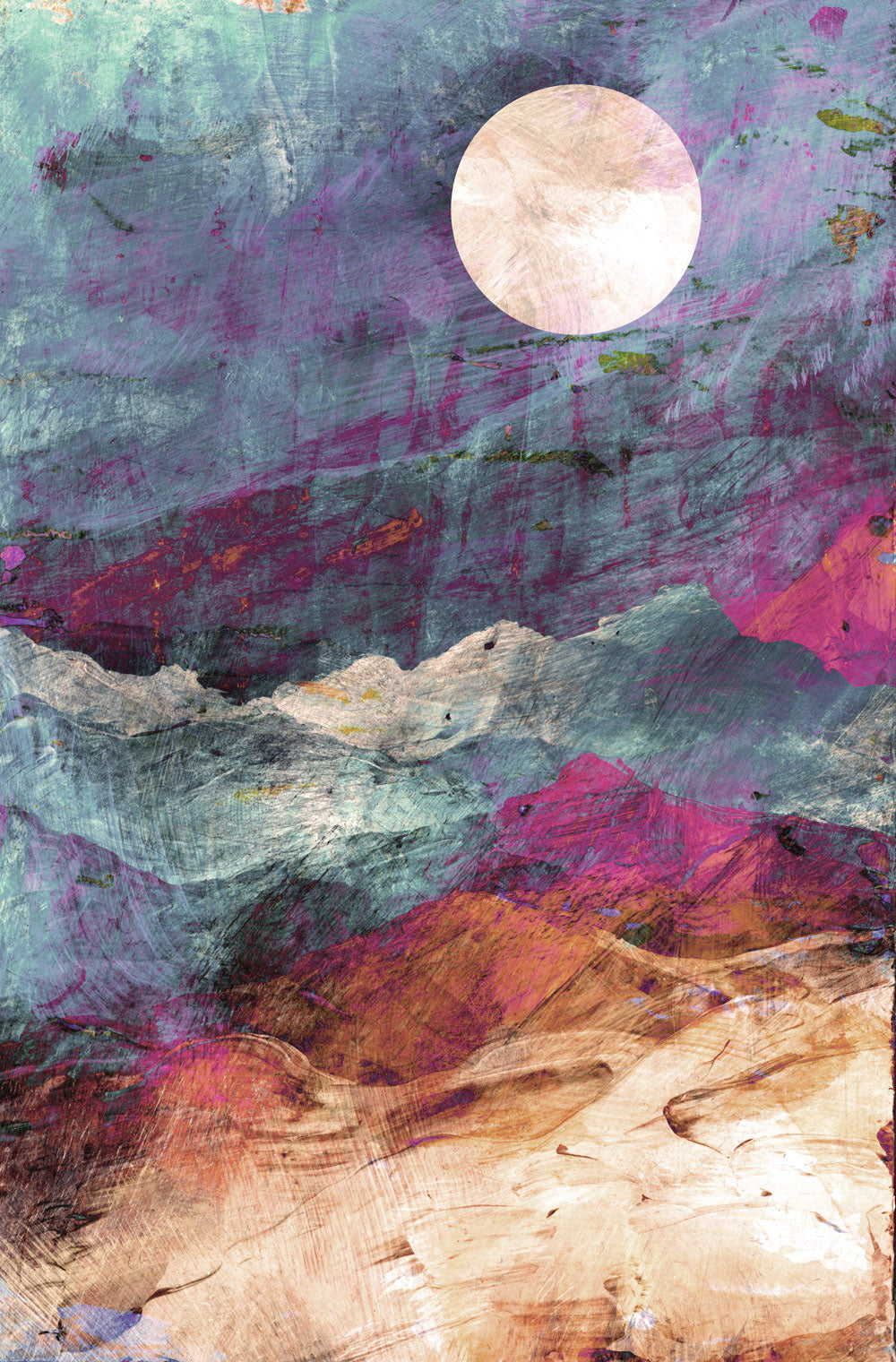The vertical painting presents an abstract and highly artistic night scene by the coast. The bottom part features aggressive, sharp-edged waves in a variety of dynamic colors such as violet, purple, dark and light browns, blue, gray, and midnight blue, suggesting a tumultuous sea. Transitioning to the middle section, the painting depicts wavy patterns in greenish-white, bluish, and reddish hues, reminiscent of the sea or ocean. The upper portion is dominated by a dark green and blue sky, interspersed with reddish splashes and scratches, creating a vivid night sky. Slightly offset to the right in the top middle, a large white circle represents a full moon, its pale white tone accented by shadows. The entire piece employs gradients and abstract styles to convey the scene, focusing on color and shadow rather than realistic details, painting a compelling, imaginative coastal landscape at night. There is no text visible in the image.